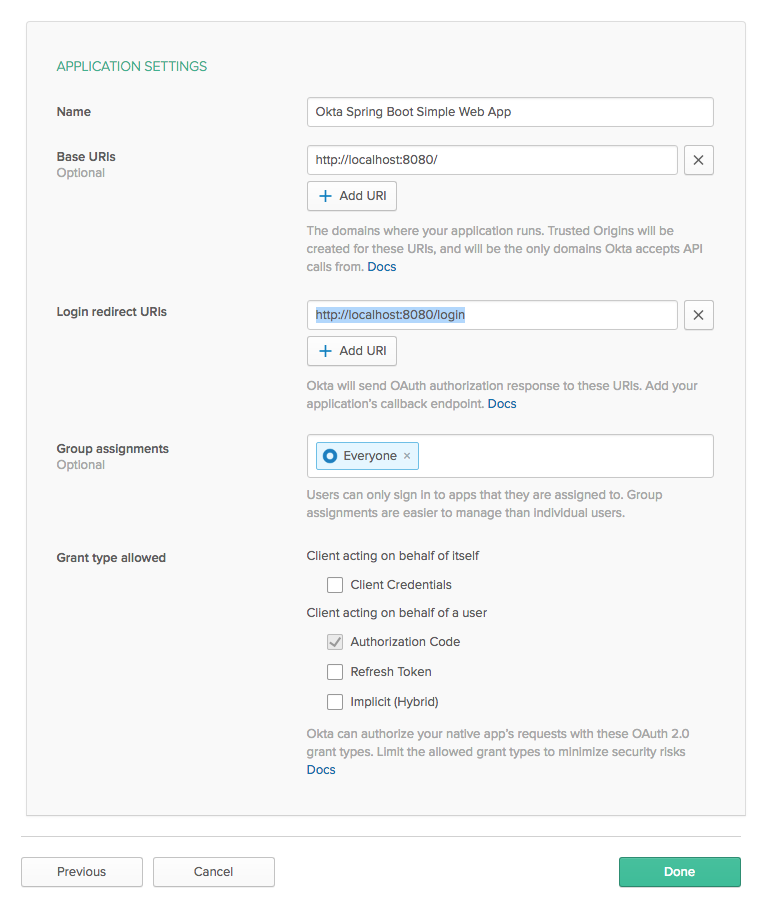**Detailed Caption for Screenshot of Application Settings Interface**

This is a screenshot of an application interface, likely related to management or configuration of other applications. At the top, there is a green header displaying "Application Settings." 

Directly below, there's a section labeled "Name" with a text field containing the title "Okta Spring Boot Simple Web App." Beneath this, the section labeled "Base URIs (Optional)" contains what appears to be a URL, despite the term URI being used. This section allows the addition of more URIs, specifying that these domains are where the application runs. Trusted origins will be generated for these URIs, ensuring that Okta accepts API calls solely from these domains. A hyperlink labeled "Docs" in blue directs users to relevant documentation.

Further down, we find the "Login Redirect URIs" section. Here, a different URI is listed, featuring an additional "/login" at the end. Multiple login redirect URIs can be added, and it is noted that Okta will route OAuth authorization responses to these URIs at your application's callback endpoint. Another "Docs" link is presented here for further guidance.

The "Group Assignments (Optional)" section follows, describing that users can only sign into applications they are assigned to. It elaborates that managing group assignments is more efficient than managing individual user access.

Below this is the "Grant Types Allowed" section, detailing options for different OAuth 2.0 grant types. For clients acting on behalf of themselves, the "Client Credentials" option is available. For clients acting on behalf of users, three options are listed: "Authorization Code," "Refresh Token," and "Implicit (Hybrid)." Okta uses these grant types to authorize native app requests and advises limiting the allowed grant types to reduce security risks.

At the bottom of the screenshot, there are three buttons: "Previous," "Cancel," and "Done," presumably for navigating or saving changes in the application settings.